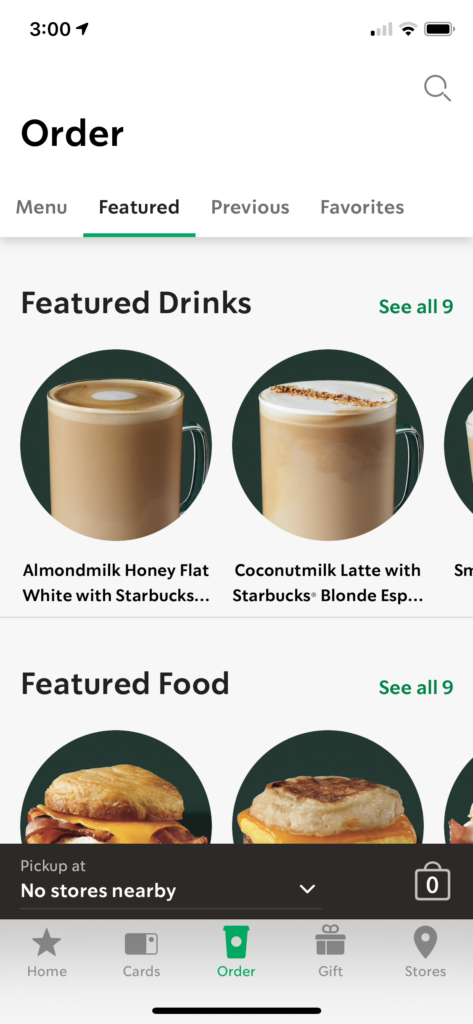### Detailed Caption

This detailed image description captures a screenshot from a smartphone featuring the Starbucks mobile ordering app. The upper section of the screenshot showcases the standard smartphone status bar with a white background. It displays the time as 3 o'clock on the left, without specifying if it’s a.m. or p.m. On the upper right corner, icons for battery status, Wi-Fi signal, and wireless connection are visible. Notably, the wireless connection is weak, as indicated by only one filled bar out of five.

Below the status bar, on the left side, the word "Order" is prominently displayed in bold black font. Beneath this, a navigation menu displays options from left to right: "Menu," "Featured" (in bold black font indicating the current page view), "Previous," and "Favorites." 

The background turns to a very light gray in the section following the navigation menu. On the left, the text "Featured Drinks" appears, and on the right, the phrase "See all 9" is written in green font, inviting users to view more options.

This is followed by two oval-shaped images of drinks, indicative of the Starbucks ordering page. The left image is partially labeled "Almond Milk Honey Flat White with Starbucks," although the full title isn’t visible. The right image is labeled "Coconut Milk Latte with Starbucks Blonde Espresso," with espresso abbreviated as "exp." Both drinks are presented in clear glass mugs, making their beautiful brown color combinations clearly visible.

Moving down, another header titled "Featured Food" appears. The images below show the top halves of two food items. The left image likely represents an English muffin with an underlayer of orange cheese, possibly American or cheddar, and what appears to be bacon. The right image is also an English muffin with an orange cheese layer beneath it, similar to the previous one.

At the bottom of the screen, the footer section has a very dark gray background displaying the message "No stores nearby" in white font under the "Pick up" section. To the right, there is a small camera icon. Below this is the phone's app-specific footer in a lighter gray, listing navigation options: "Home" (indicated by a star for the Starbucks logo), "Cards," "Order" (highlighted in green), "Gifts," and "Stores."